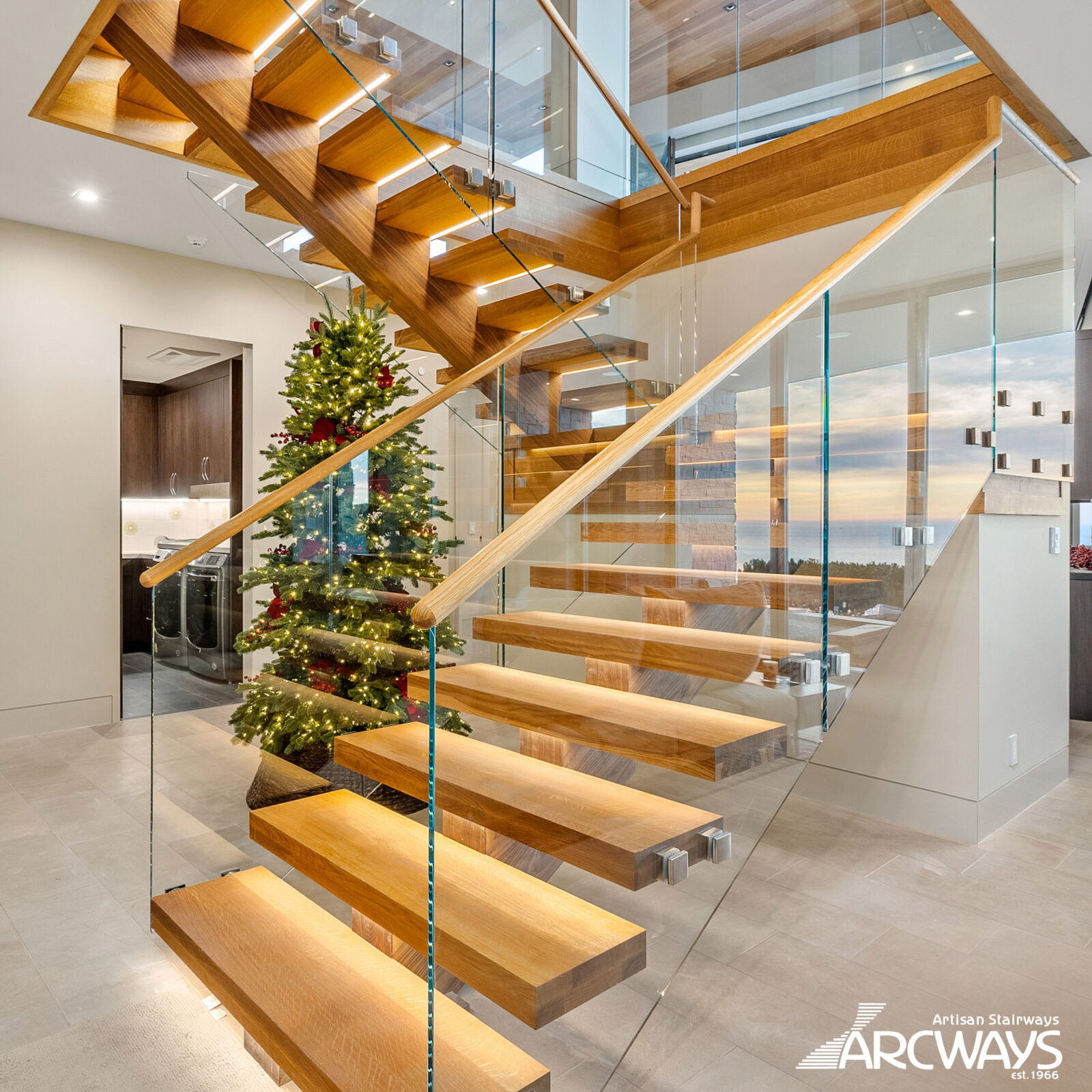The photograph showcases a modern, indoor scene featuring a striking, double-set wooden staircase. Each flight of the staircase comprises about eight light wooden steps, separated by a long central beam, giving a floating illusion. The stairs are bordered by sleek glass panels that are topped with wooden railings. To the left of the first staircase and underneath the second is a tall Christmas tree adorned with fairy lights and red ribbons, adding a festive touch. The background reveals a glimpse of a kitchen, suggesting an open floor plan. The overall design is airy and bright, emphasized by the natural sunlight streaming in. The bottom right corner of the image contains text that reads "Artisan Stairways, Archways, established since 1966," indicating that this is an advertisement.